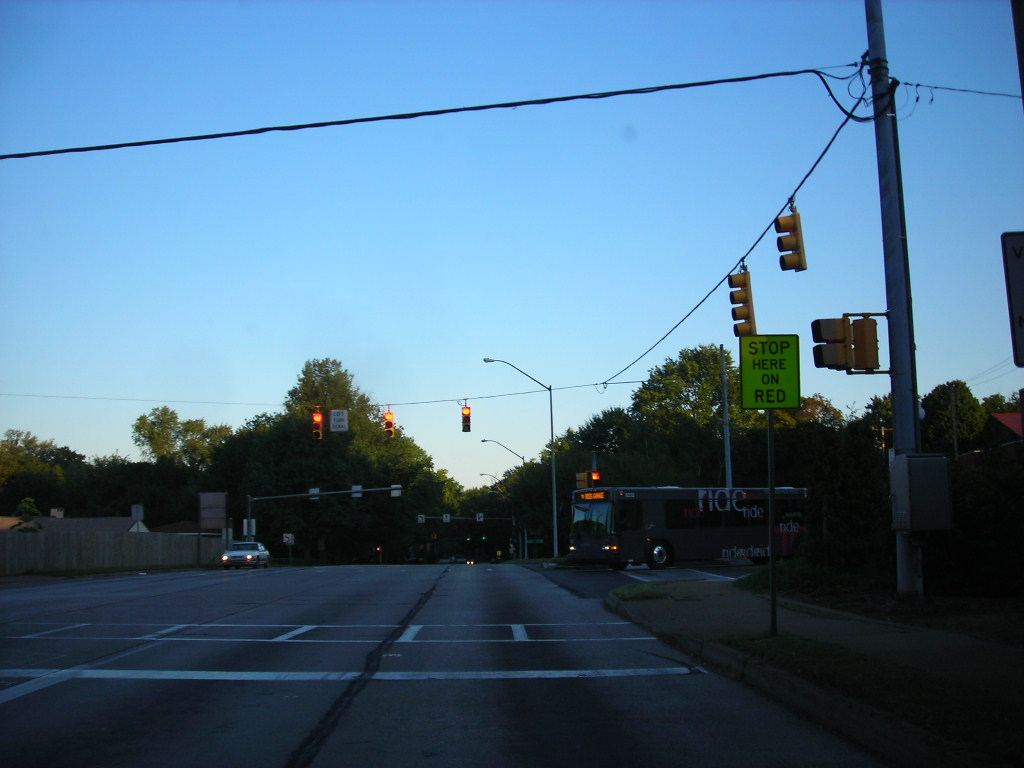A high-resolution photo captures the view from the front of a vehicle, possibly from a dashcam or a camera mounted atop the vehicle. The vehicle is halted at a stoplight in the far right lane of a multi-lane road. Though no part of the vehicle is visible, the composition places the viewer directly at the intersection. To the left, a well-maintained curb and sidewalk edge the road, accompanied by a silver pole with a road sign reading "STOP HERE ON RED" situated on a small grassy strip. A horizontal white stop line is conspicuous just to the left of the sign. 

In the distance, three red traffic lights dangle from an overhead wire, signaling the stop. The intersection reveals various vehicles halted in their lanes; prominently, a large brown bus with a digital display showcasing orange text and with its headlights illuminated. It pauses perpendicular to the direction of the viewer’s vehicle. Additionally, a small white car is positioned to the left in the background, also stationary.

The bright blue sky above contrasts with a web of power lines that traverse the upper section of the photograph, adding to the urban atmosphere. The scene is imbued with a sense of pause and order, depicting a typical moment at a busy city intersection.